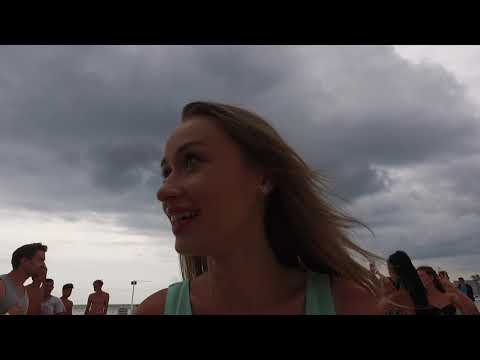In this image, we see a young woman in her late 20s taking a selfie, possibly a video. She has long, dark blonde hair and is wearing a green tank top. Her skin is fair, and she is smiling while looking off to her right, as if engaging with someone just off screen. The lighting is poor, making the image somewhat dark and giving it a grainy quality. Surrounding her are several people around her age who are milling about and talking amongst themselves. The cloudy sky overhead suggests impending stormy weather. While the setting isn't clearly identifiable due to the low angle of the shot, it gives the impression of an outdoor event or a recreational venue, possibly even a beach during a spring break-type event.